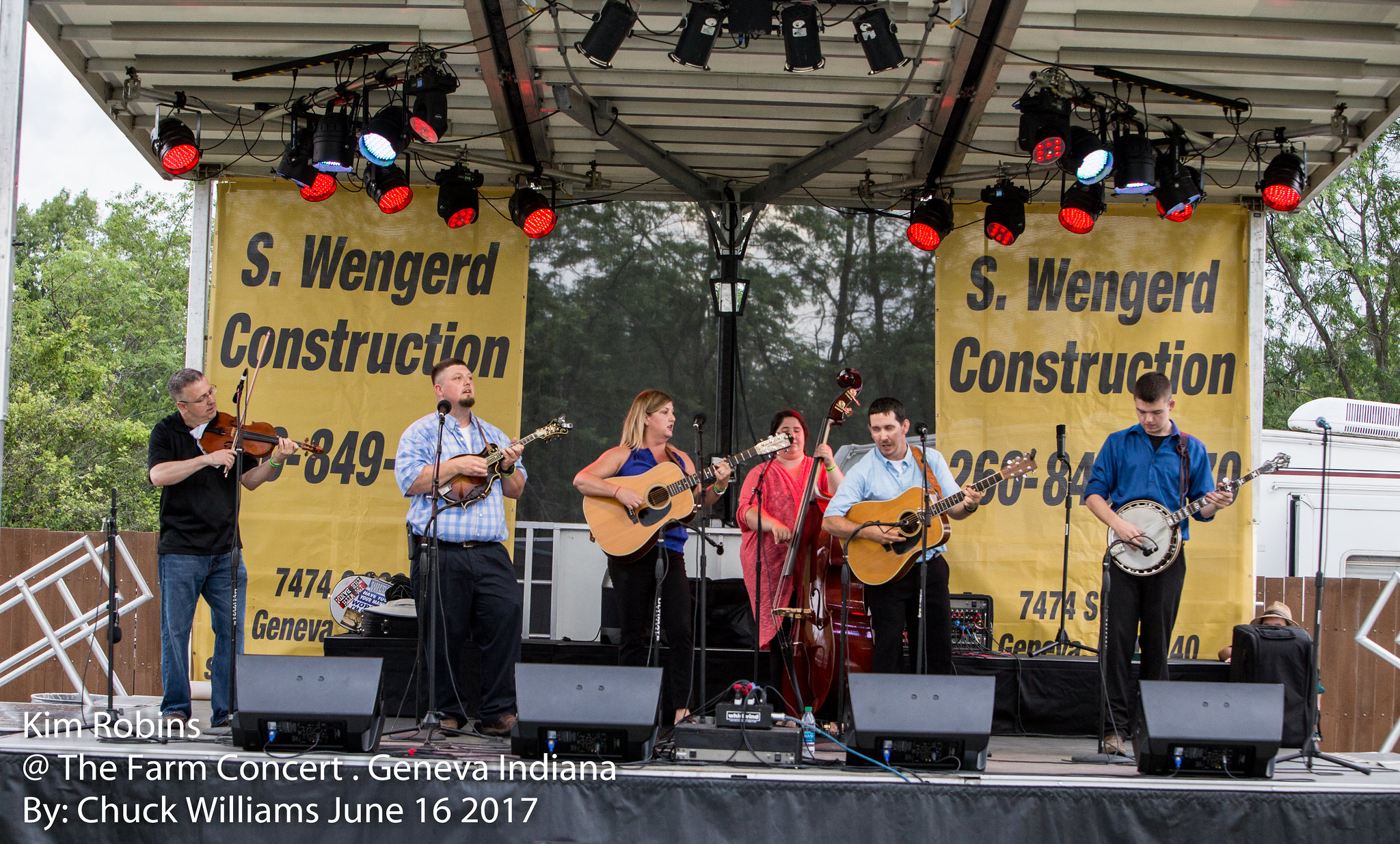In this detailed image, a bluegrass folk band performs on stage at the Farm Concert in Geneva, Indiana, on June 16, 2017. Captured by Chuck Williams, the photograph features four men and five women, each with a string instrument. From left to right, we see a man in a black shirt playing a violin, beside him, another man in a light blue plaid shirt playing what appears to be an acoustic guitar. Next, a woman holds another acoustic guitar, with a woman behind her playing a cello. Another man handles an acoustic guitar, positioned next to a man on the far right in a blue shirt, playing a banjo. Behind them, a prominent yellow sign advertises "S. Wengard Construction" along with a phone number. In the bottom left corner, the caption reads, "Kim Robbins at the Farm Concert, Geneva, Indiana by Chuck Williams, June 16, 2017," indicating that Kim Robbins may be a featured performer or part of the band.